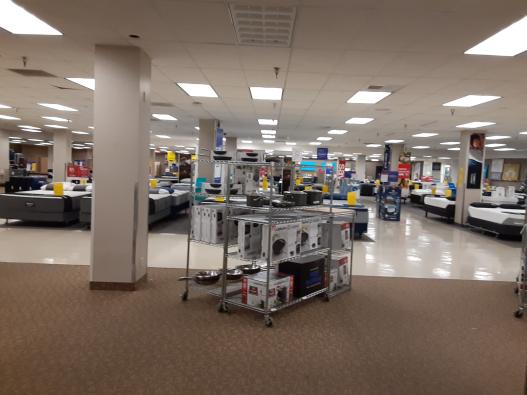The image depicts the interior of a department store, potentially resembling a JCPenney or Macy's, characterized by its mixed flooring of brown, paisley-patterned carpet and white vinyl tiles. The store's ceiling features a grid layout with various blocks removed to accommodate lights and air vents. Scattered throughout the space are numerous columns with white finishes and wooden trims at the base.

Prominent in the center are portable metal shelves on wheels, laden with a variety of cookware, including black pots with silver lids and other cooking utensils. Flanking these displays on both the left and right sides are numerous mattresses, some with gray box springs and black labels. These mattresses are set up for customers to try, complete with strips of fabric covering the bottoms to keep them clean from shoes. Yellow tags, enclosed in plastic, provide pricing and sales information.

A notable column rises from the carpeted floor to the ceiling, further dividing the space and adding to the organized yet bustling atmosphere of the store. The overall setup suggests a diverse retail environment offering a wide range of household items, from kitchenware to bedroom furniture.